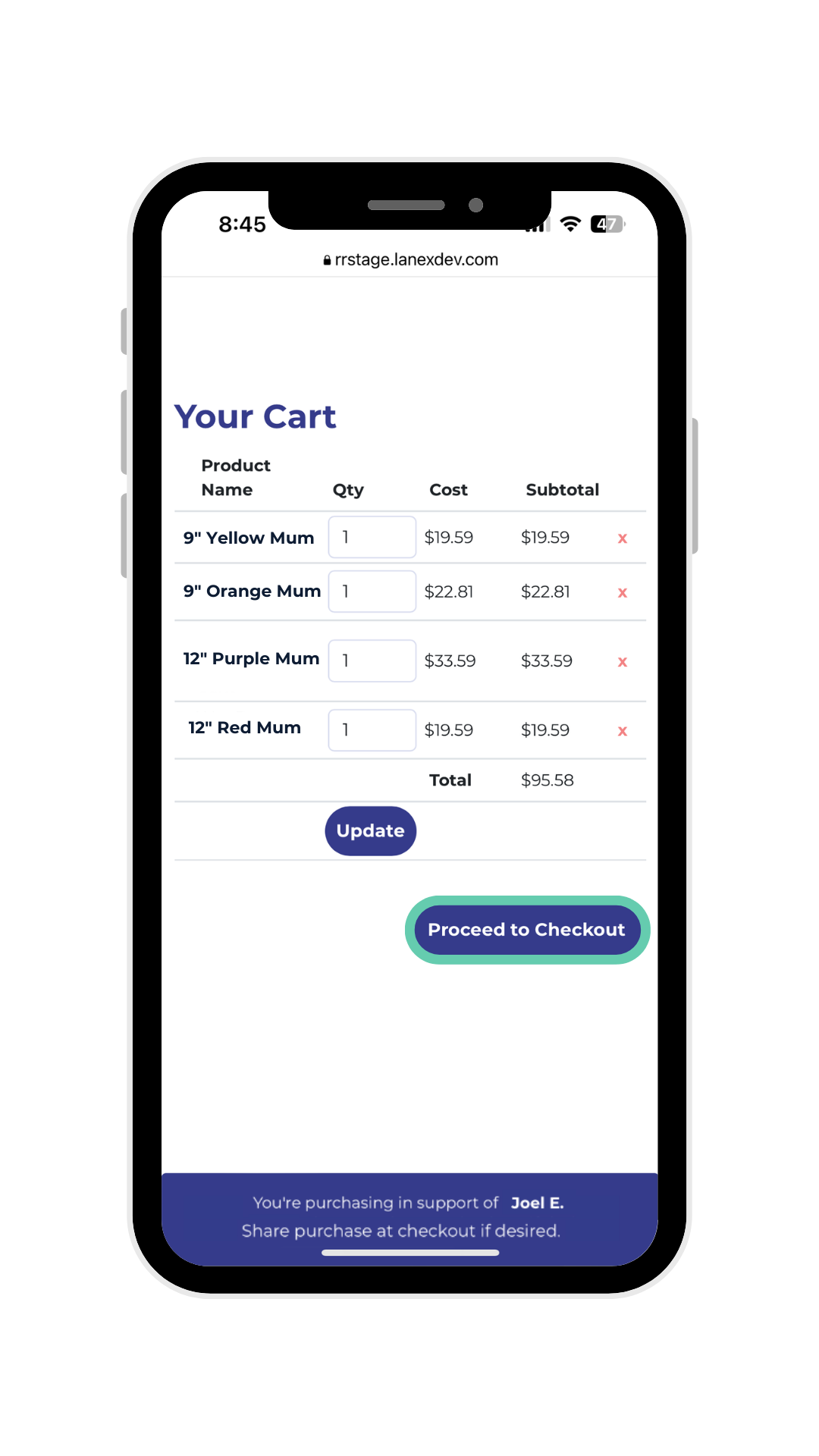The image displays an Android interface with a daylight theme, featuring a white background and predominantly black text. At the top of the screen, a heading titled "Your Cart" appears in blue text. The interface is accessed via a web browser, indicated by the URL rrstage.lanexdev.com displayed at the top of the screen. The unfamiliar URL suggests it may be a development or staging site.

Below the "Your Cart" heading, a detailed table itemizes the products currently selected for purchase. The columns in the table are labeled: Product Name, Quantity, Cost, and Subtotal. The listed items are:

1. 9-inch Yellow Mom - Quantity: 1, Cost: $19.59, Subtotal: $19.59
2. 9-inch Orange Mom - Quantity: 1, Cost: $22.81, Subtotal: $22.81
3. 12-inch Purple Mom - Quantity: 1, Cost: $33.59, Subtotal: $33.59
4. 12-inch Red Mom - Quantity: 1, Cost: $19.59, Subtotal: $19.59

The total expenditure amounts to $95.58.

Adjacent to the table, there is a blue, rounded rectangle button labeled "Update," which likely allows users to modify the quantity of the items in the cart by entering new values in the associated text boxes before clicking the button. Below and slightly to the right of the "Update" button is another blue, rounded rectangle button labeled "Proceed to Checkout," guiding the user to finalize their purchase.